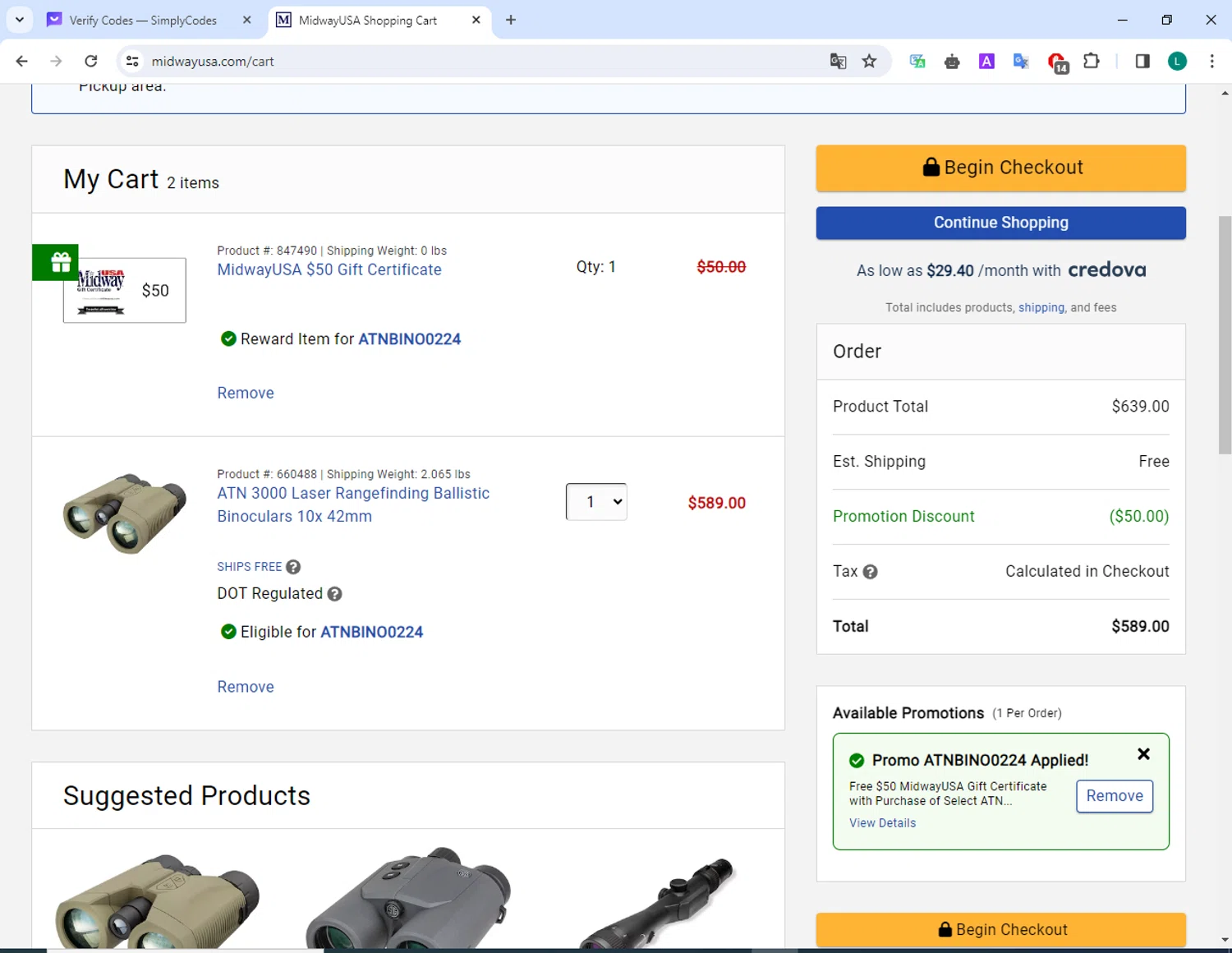Screenshot from MidwayUSA Shopping Cart:

The screenshot captured from MidwayUSA.com showcases a user's shopping cart. The cart contains two items: a $50 MidwayUSA gift certificate and a pair of laser range-finding ballistic binoculars priced at $589. At the top of the cart section, displayed in a prominent bold black font, it reads "My Cart - 2 items."

Below the listed items, several suggested products are visible, including what appears to be more binoculars and a flashlight. To the right of the product listings, there are functional buttons to navigate the shopping process. The "Begin Checkout" button is highlighted in yellow with black text, while the "Continue Shopping" option is presented as a blue bar with white text.

The cart summary includes details about the product total, a note indicating free shipping, a promotional discount of $50 (bringing the total down to $589), and a reminder that taxes will be calculated at checkout. There's also an indication that a promo code has been applied. Another "Begin Checkout" bar is located at the bottom of the screen for convenience.